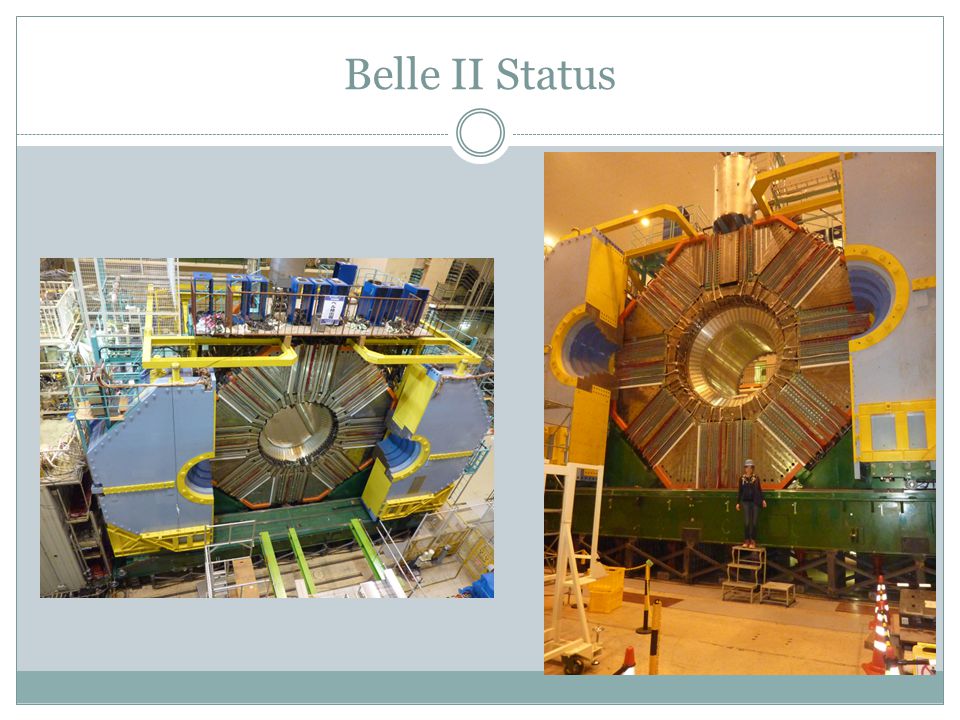The image is divided into two sections, both under a banner that reads "BELL II STATUS" in capitalized, blue letters on a white background, with "II" spelled in Roman numerals. The picture on the left showcases a large, complex circular metallic structure composed of interconnected steel frames, turbines, and a grid design, suggesting an industrial or scientific setting within a factory. Predominantly silver, blue, and yellow hues color this intricate equipment. On the right, a person stands beside the structure for scale, revealing its immense size—about 20 times bigger than a human, requiring the person to stand on a stepping stool to reach partway up. This side view emphasizes the massive scale and intricate design, likening it to a giant metallic portal or pentagon with a central circle potentially designed to accommodate another element. The use of industrial colors like bronze, silver, blue, and yellow adds to the impression of a high-tech research facility. The overall composition vividly contrasts the detailed machinery and the human scale, underscoring the impressive engineering feat.